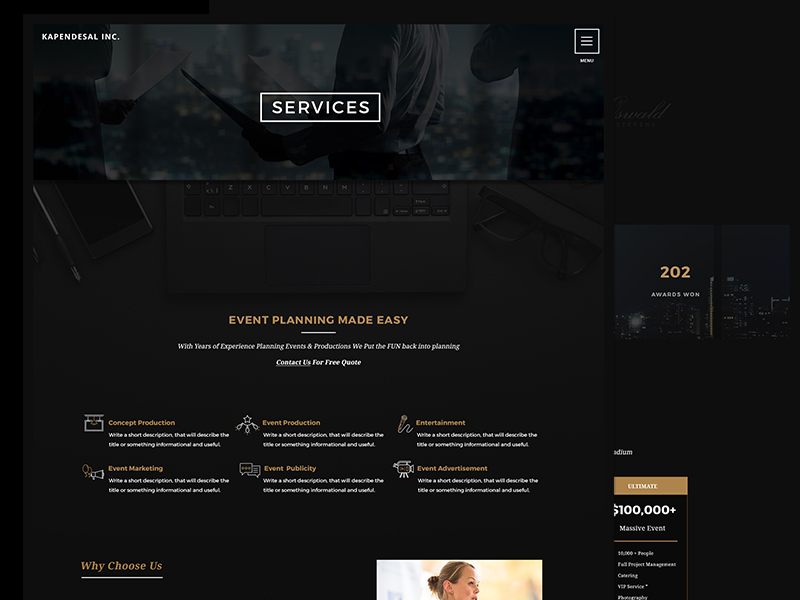The image features a predominantly black background in the top left corner with the text "Caspian DeSalle Incorporated" displayed prominently. Below that is a white box with the word "SERVICES" in bold, capital letters. Behind this overlay, there is a photograph of an individual carrying a stack of papers, alongside a desk that is neatly arranged with a smartphone, an ink pen, a laptop, and a pair of glasses. The text "Event Planning Made Easy" stands out, highlighting the firm's expertise. Additionally, the image notes an impressive achievement of having won 202 awards. Below, there are six small, somewhat blurry sections that list detailed offerings including concept production, event marketing, event production, event publicity, entertainment, and event advertisement. An additional text block prompts, "Why Choose Us," followed by a mention of "$100,000+" in value or savings, underlining the economic advantage of their services.